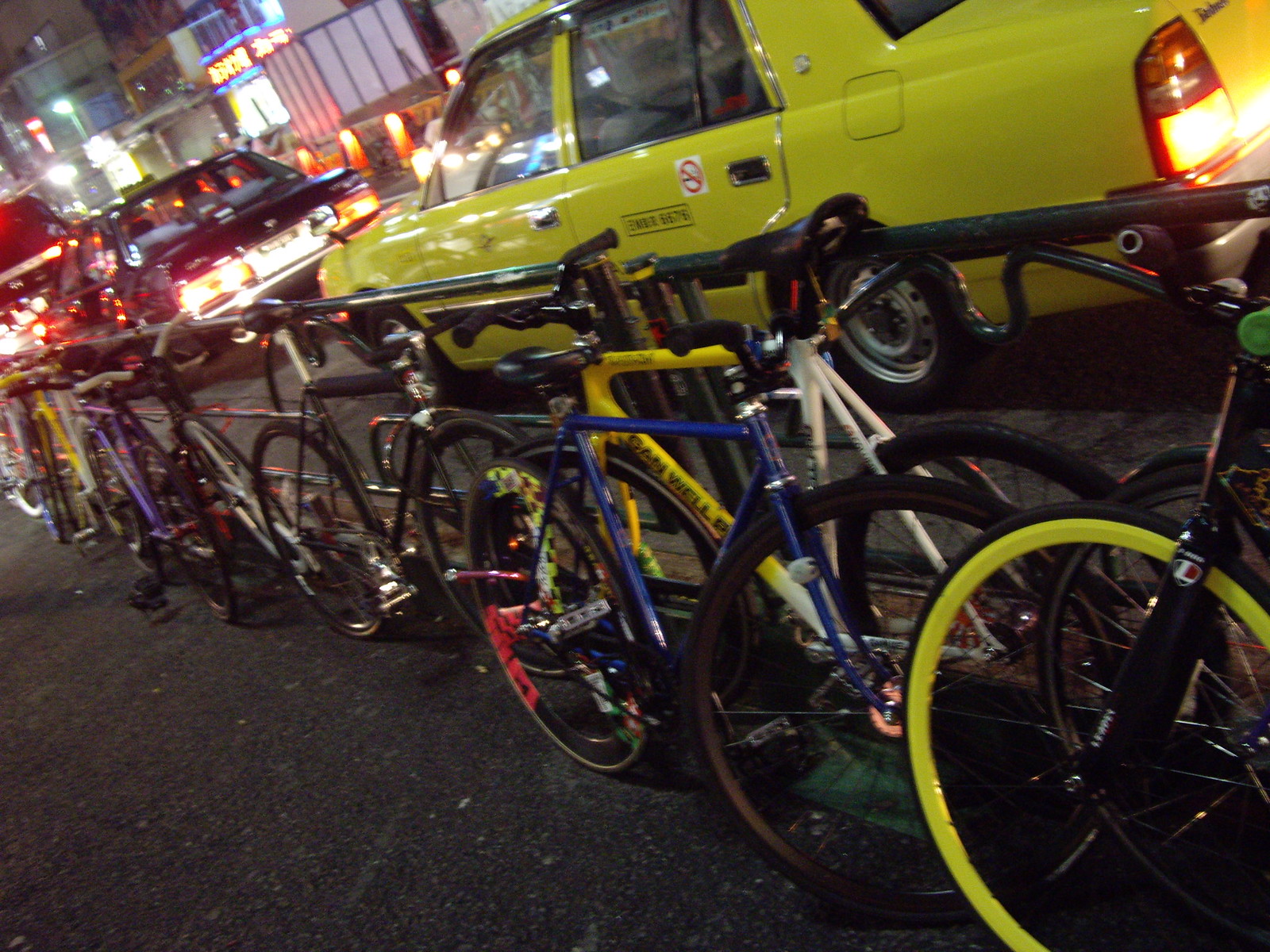This is a nighttime photograph capturing a busy city street in a foreign country. The image prominently features a row of bicycles locked to a long black bike rack running parallel to the street. The bikes are of various types and colors, including blue, yellow, white, and neon, with different colored tires such as yellow and black. Beyond the bike rack, oncoming traffic is visible, including a prominent yellow taxicab and another darker vehicle. The scene is illuminated by bright city lights and neon signs on buildings, contributing to the bustling atmosphere. The photo's lower third shows the asphalt of the street, emphasizing the urban setting.